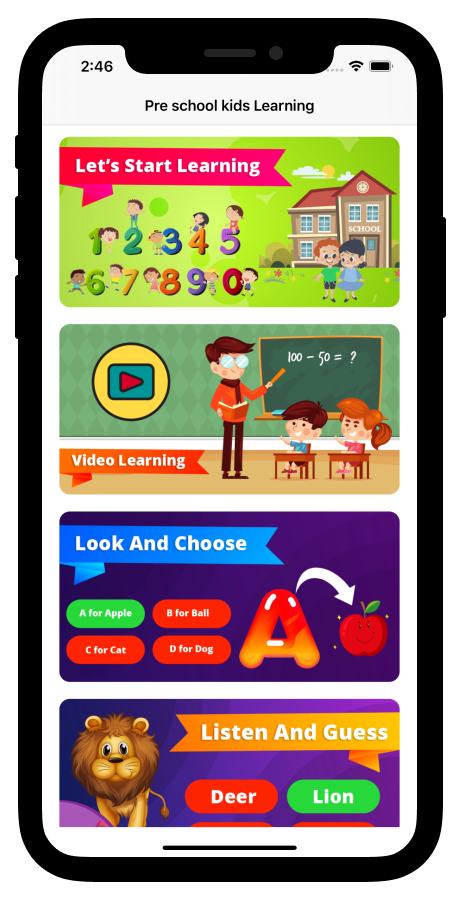The image portrays a smartphone displaying a preschool learning app. In the upper left corner, the time is shown as 2:46. The header at the very top of the screen reads "Preschool Kids Learning." The app screen is organized into four vertical rectangles, each containing different educational content.

- The top rectangle features a green background and a colorful illustration of a school with children and the numbers 0 through 9, each accompanied by a small child. A pink banner with the text "Let's Start Learning" spans across the top.
- The second rectangle is focused on "Video Learning" and displays an image of a teacher standing by a blackboard, with two students seated at desks.
- The third rectangle is labeled "Look and Choose" and shows the letter 'A' with an arrow pointing to an apple, indicating a learning activity where children select the correct answer.
- The bottom rectangle presents a "Listen and Guess" activity. It illustrates a lion with multiple ovals containing words, where users have to pick the correct word corresponding to the image of the lion.

Each rectangle is designed to offer engaging and interactive educational experiences for preschool children, promoting early learning in a fun, visual format.